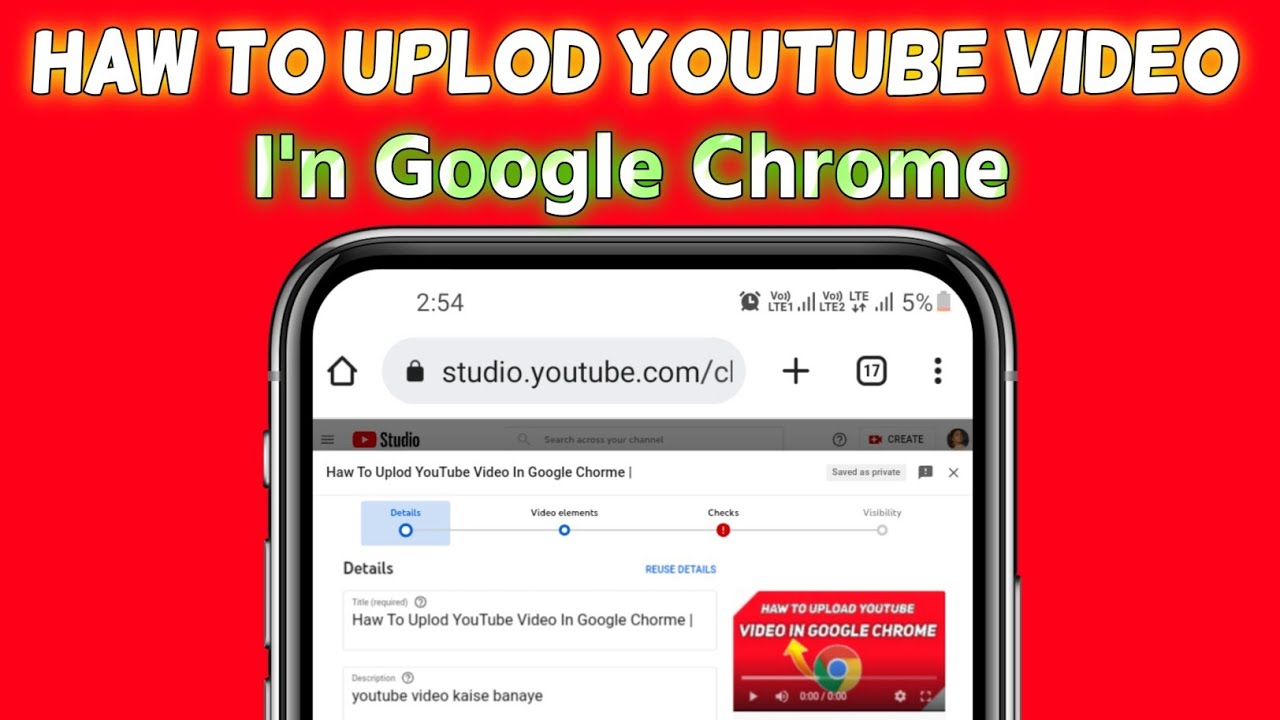The image appears to be a screenshot or thumbnail from a YouTube instructional video. The background is a bold red, providing a striking contrast to the elements in the foreground. Central to the composition is the upper half of a smartphone, featuring the interface of the YouTube Studio app indicated by the text "studio.youtube.com" displayed on the screen. This suggests that the video is aimed at content creators navigating their YouTube accounts. Above the phone and set against the red backdrop, white text prominently reads "How to Upload YouTube Video on Google Chrome." However, several typographical errors are evident: "How" is misspelled as "HAW," "upload" is missing the letter 'a', and "in" Google Chrome is incorrectly written as "I'N." These mistakes hint that the creator's first language might not be English. Despite these errors, the intent of the video remains clear—to guide users through the process of uploading a YouTube video using Google Chrome.